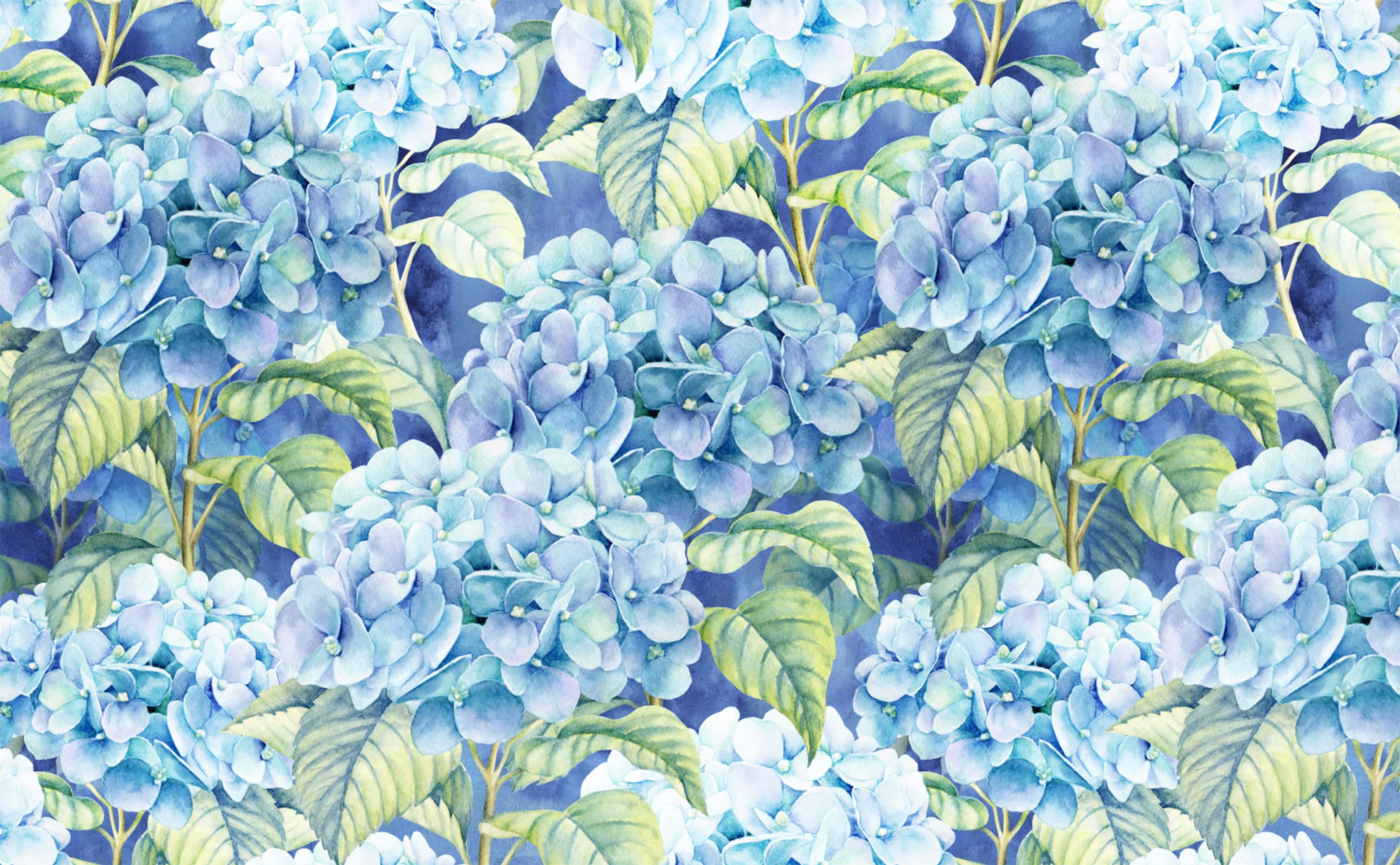This image depicts a vibrant watercolor painting of blue and purple hydrangeas, characterized by varying shades of blue, from pale to deep, and purplish tints. The clustered flowers are accented by large green leaves in different hues, creating a vivid, almost pattern-like design that could be used for curtains or wallpaper. The arrangement is repeated across the canvas, starting with light blue flowers in the lower left and transitioning to darker purple hues, before circling back to light blue at the top. The green stems and leaves intertwine, adding texture and depth, while the background features multiple shades of blue, enhancing the overall visual appeal and making the flowers stand out. This piece has areas of light and shadow, adding an artistic effect that suggests a natural setting, perhaps a wildflower field, rather than a tended garden.